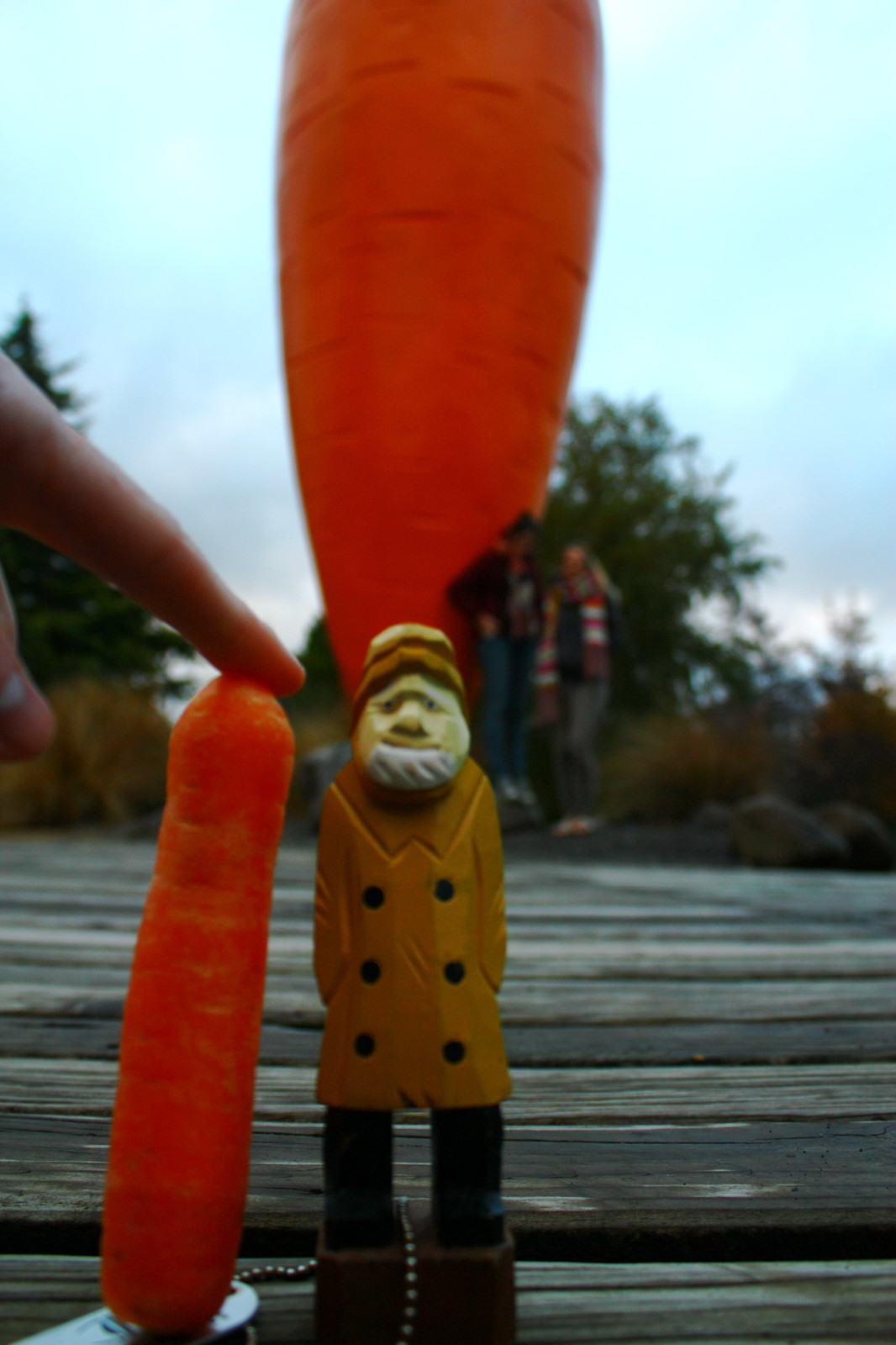This is an image of a small, intricately carved wooden figurine of an old man, prominently positioned on a wooden dock or walkway. The figurine, which appears to represent a garden gnome, is dressed in a yellow coat with black buttons, a matching yellow hat, and thick black boots. He sports a white beard and has a Caucasian complexion. A finger from the left side of the image is holding up a carrot next to the figurine, drawing attention to its diminutive size in comparison to the finger. In the blurred background, there are a few people standing next to what seems to be the bottom half of a giant carrot against a backdrop of trees and bushes. The photo captures a clear blue sky, enhancing the outdoor setting. The close-up perspective makes the figurine appear larger than it actually is, making it the main focal point of the image.